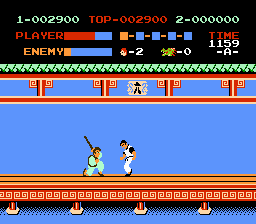The screenshot features a classic fighting video game distinguished by its pixelated graphics, suggesting its vintage origin. The game appears to involve two characters, with one potentially being an NPC (Non-Player Character) and the other controlled by a player. This presumption arises from the interface displayed at the top of the screen, which occupies about a quarter of the image against a black background. Here, player stats are clearly labeled, accompanied by life bars for both the player and the enemy, indicating the remaining health for each combatant. The game's aesthetic and character design evoke a karate theme, enriched by traditional martial arts elements that heighten the nostalgic atmosphere of the gameplay.